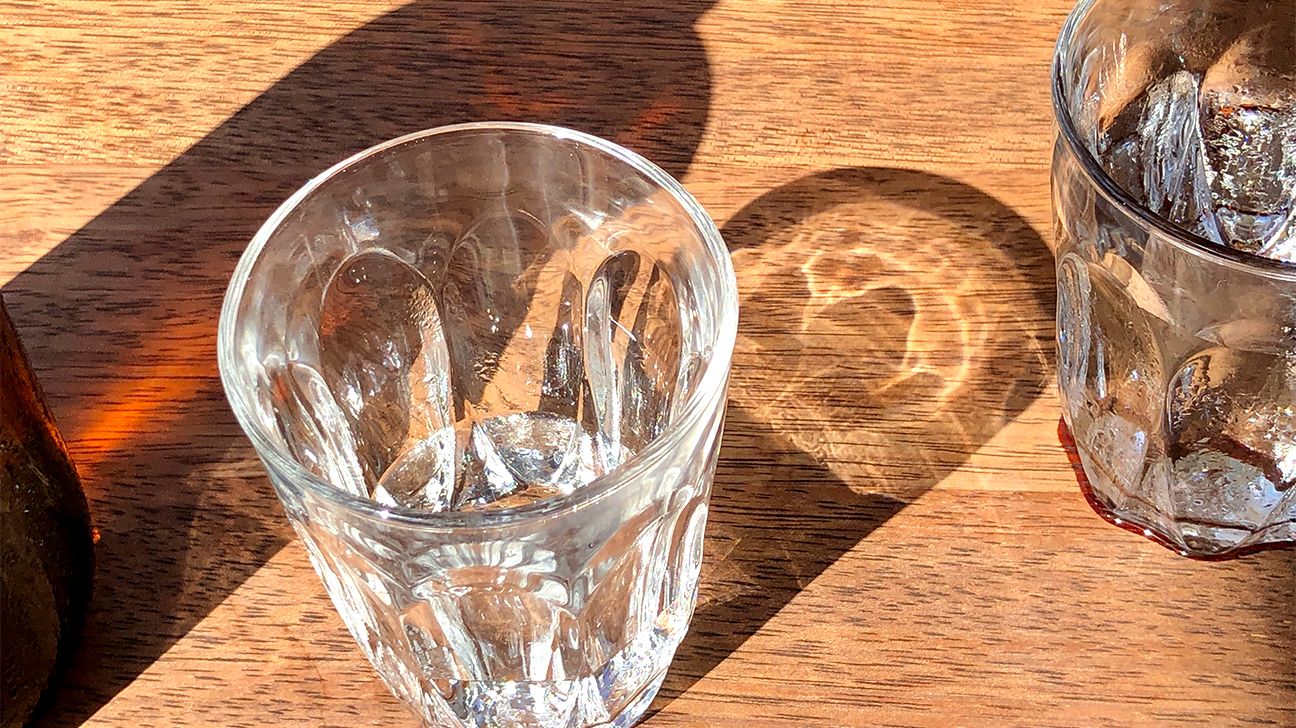This close-up photograph features two transparent glasses and a partially-visible bottle on a light brown wooden table. To the right, half of a glass filled with ice and a small amount of water is shown, with the top of the liquid level visible. Towards the center, there is an almost empty glass with a visible shadow on the wooden surface. On the left, only the bottom of a bottle is faintly visible, but its silhouette is distinguishable, casting a shadow on the wood grain below. The glasses resemble mini shot glasses or whiskey-sour glasses, emphasizing the bright light casting distinct shadows and reflections across the scene.